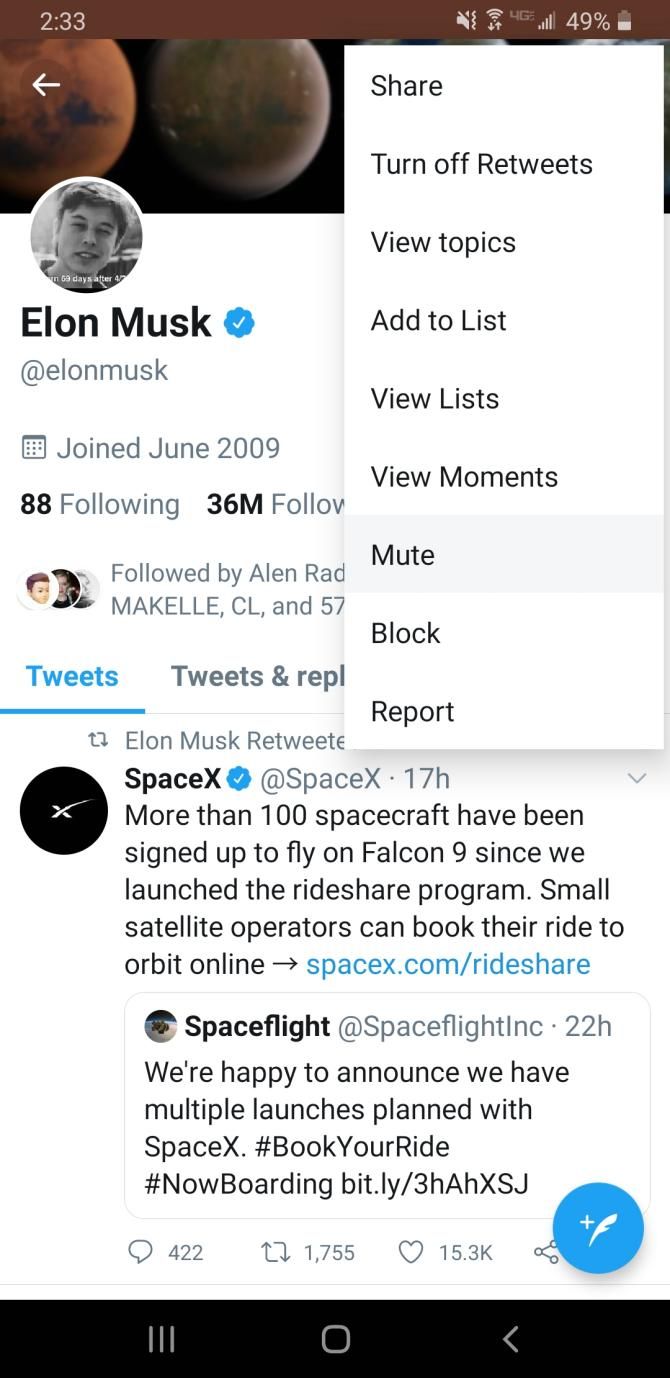The image portrays a screenshot of a smartphone displaying a Twitter page. The phone screen shows a time of 2:33 with three bars of signal strength and a battery level at 49%. The top part of the screen displays options such as "Share," "Turn off Retweets," "View Topics," "Add to List," "View List," "View Moments," "Mute," "Block," and "Report."

The screenshot is focused on Elon Musk's Twitter profile, which features a blue verification checkmark. The bio section reads "@elonmusk," with a note that Elon Musk joined Twitter in June 2009. The profile further shows that Elon Musk is following 88 accounts and has 36 million followers. Information about mutual followers is partially cut off.

Below the profile information, various tab options like "Tweets" and "Tweets & Replies" are available. The highlighted tweet mentions, "More than 100 spacecraft have been signed up to fly on Falcon 9 since we launched the rideshare program. Small satellite operators can book their ride to orbit online." A link to "spacex.com/rideshare" is provided in blue text, following a black separator line.

Another tweet from the account @SpaceflightInc, posted 22 hours ago, states, "We're happy to announce we have multiple launches planned with SpaceX." It includes hashtags "#BookYourRide" and "#NowBoarding," along with a shortened URL "bit.ly/3hahxsj."